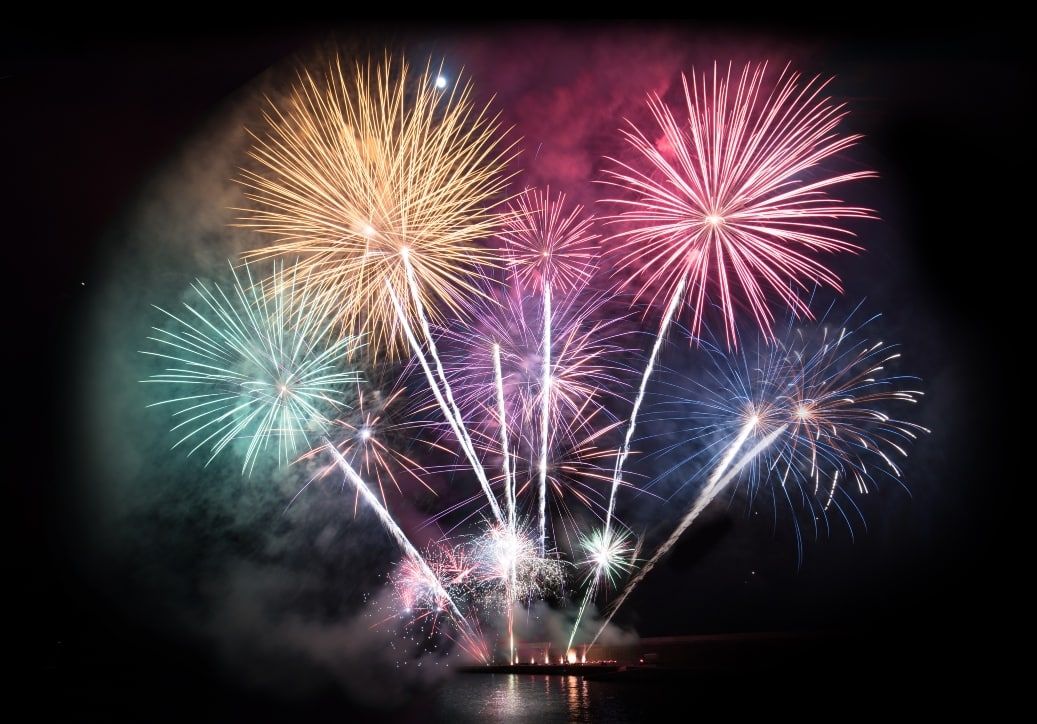This captivating long-exposure photo, taken at night, features a dazzling display of fireworks over a calm body of water. The scene is set against a stark black background, which makes the vibrant colors of the fireworks stand out dramatically. The fireworks, deployed from a large barge on the water, include a green one on the left, a yellow one at the top left, a pink one at the top right, and a blue one on the bottom right. Additionally, there are smaller fireworks in hues of purple, pink, and green scattered throughout the image. A thick smoke, tinted by the colors of the fireworks, lingers in the air, adding depth to the spectacle. At the top of the scene, above the yellow firework, a bright white moon and a few stars can be seen, highlighting the serene and clear night. The water beneath is calm, with no visible waves, suggesting a tranquil and windless evening. The overall scene showcases a beautifully orchestrated nighttime celebration on a small island or barge, highlighted by the colorful and varying bursts of fireworks illuminating the sky.